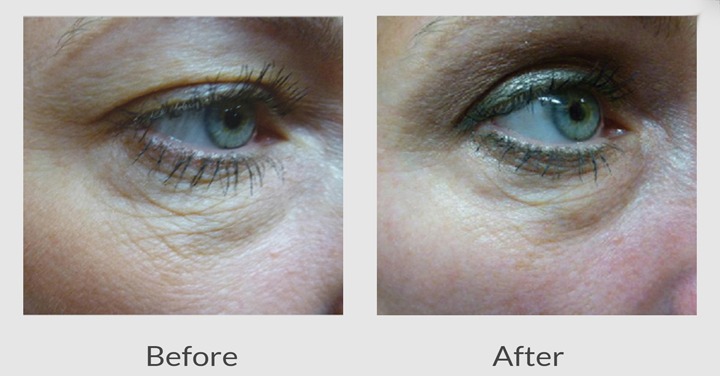The image consists of two side-by-side, close-up photos of a woman's eye, labeled "before" and "after" underneath each respective picture. In the "before" photo on the left, her blue eye appears partly covered by drooping skin from the upper eyelid, which causes the eyelid to sag noticeably. The area around her eye shows prominent bags and wrinkle lines, with some redness visible in the corner of the eye. Her eyelashes are visible, and she appears to have some makeup on. In the "after" photo on the right, following what appears to be an eyelid lift surgery, her eyelid is markedly tighter, no longer sagging over her eye, and her bags and wrinkles around the eye are significantly reduced. This has allowed her eye to open wider, presenting a rejuvenated and fresher appearance. The redness is absent, and the overall skin around her eye is smoother. Her blue eye, eyelashes, and makeup are still visible in this photo, emphasizing the successful result of the surgery.